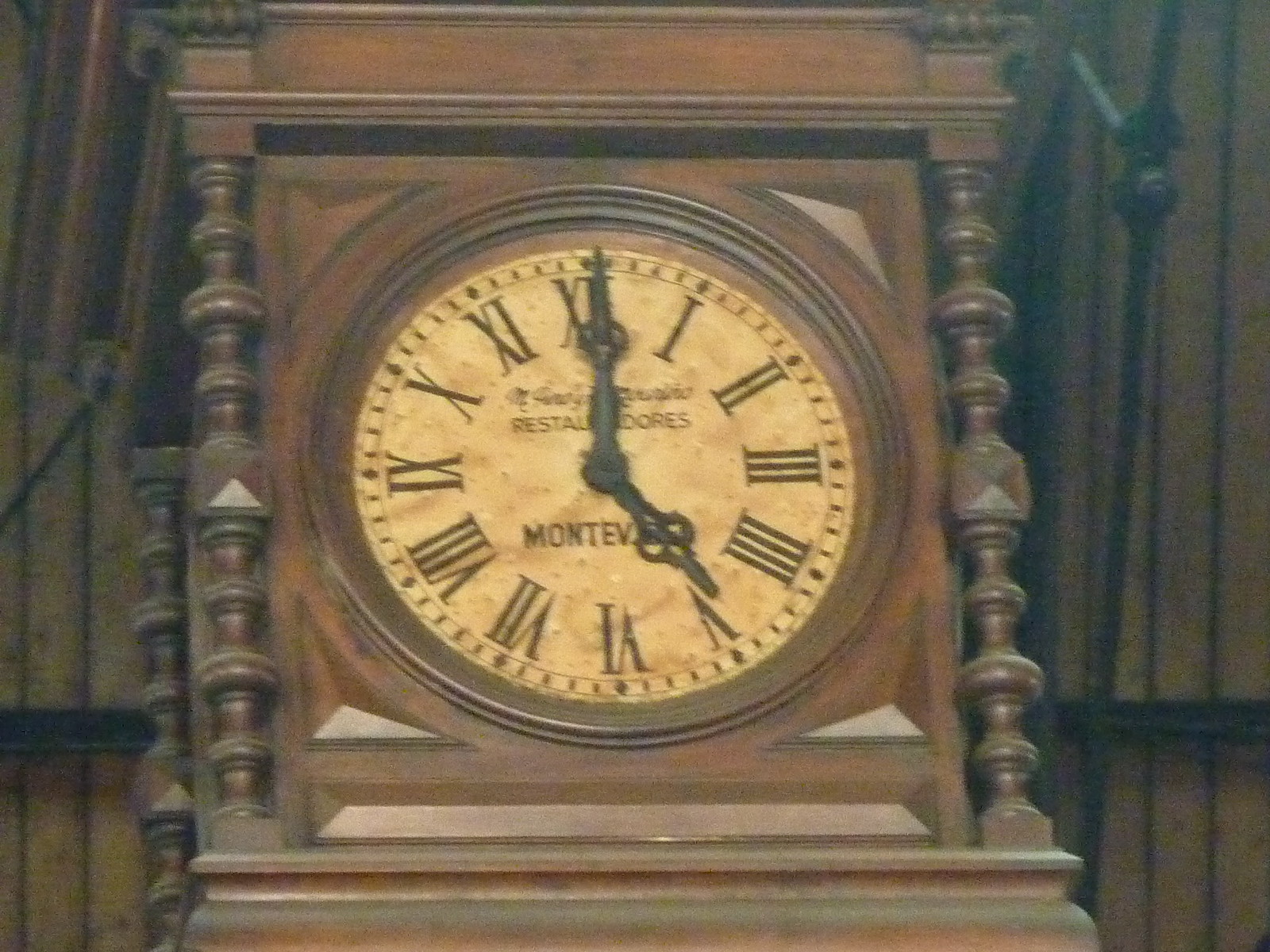The image features an ornate, antique wooden clock, likely from the early 1900s, set against a hazy, black background that could either be wood or fabric, though it is difficult to determine. The clock, designed in a mantle clock style, is square-shaped and prominently positioned in the center of the image. It showcases finely carved and turned dowels, or spindles, on either side of the face, enhancing its ornate appearance. The wood, possibly walnut, has a rich, old patina that suggests significant age, even showing hints of dust.

A darker brown, beveled and raised outline frames the clock face, which is parchment-colored and faded, indicative of its age. The clock dial features Roman numerals and two ornate hands with a design including four circles near the tips, contributing to its intricate detail. The hour hand is approaching 5 o'clock, partially obscuring the inscription, which reads "Montev," though additional text is hidden. The overall construction of the piece includes four wooden pillars at each corner, hinting at the clock’s substantial size and well-crafted design.